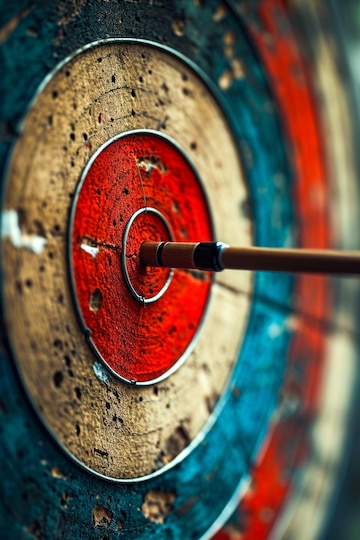This photo is a close-up of a well-worn dartboard, sharply focused on the center portion, or bullseye. The bullseye itself is a vibrant red circle, with a dart precisely embedded in its center. Surrounding the red bullseye is a series of colored rings: a white ring, followed by a larger blue ring, and multiple concentric rings in red, brown cork, and teal. The dartboard is visibly aged and heavily punctured by numerous previous hits, especially apparent in the cork area, which shows many holes of varying sizes. The image captures the central colors clearly, but the farther right side of the board and its outer rings become slightly blurred, yet still discernible. Overall, it highlights not only the target's color patterns but also its character from extensive use.